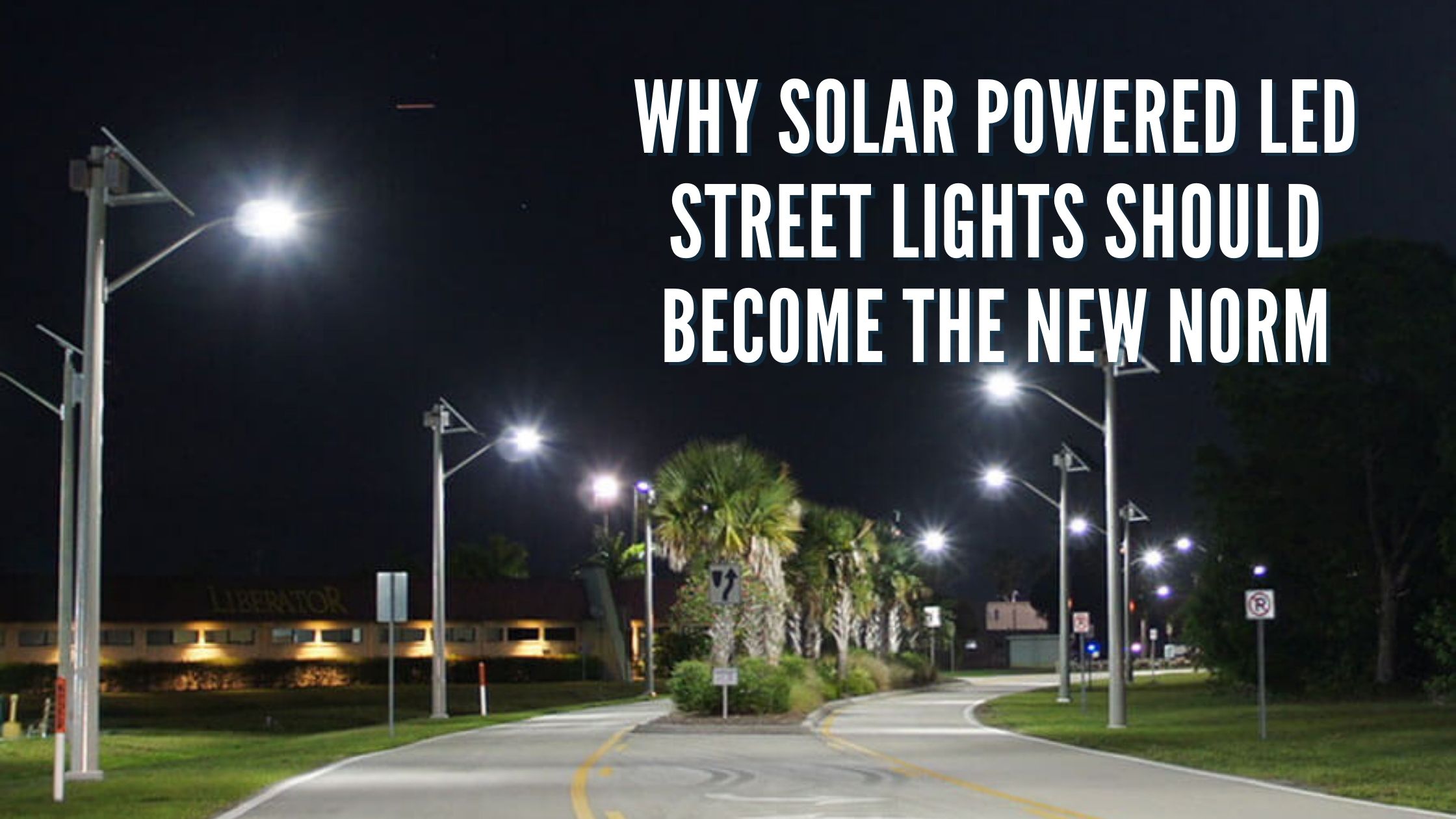The image is a detailed, color photograph set against a predominantly black night sky, taken in a narrow, wide, horizontal format. The scene captures a nighttime street in a town, illuminated by multiple streetlights, possibly six to eight, which line both sides of a light gray, two-way road. The streetlights cast a warm glow over well-manicured green lawns that flank the road. Down the center of the street runs a median adorned with mature palm trees and neatly trimmed bushes.

In the background, there are various buildings, including what appear to be an apartment complex and possibly other structures farther in the distance. The road features clearly marked yellow lines, contributing to the sense of realism in the scene. Prominent white, bold, all-caps text overlays the top right corner of the image, reading, "Why solar-powered LED streetlights should become the new norm," suggesting that the photograph is intended for an article advocating the adoption of energy-saving LED streetlights. The overall style of the image blends photographic realism with elements of typography and graphic design to emphasize its message.